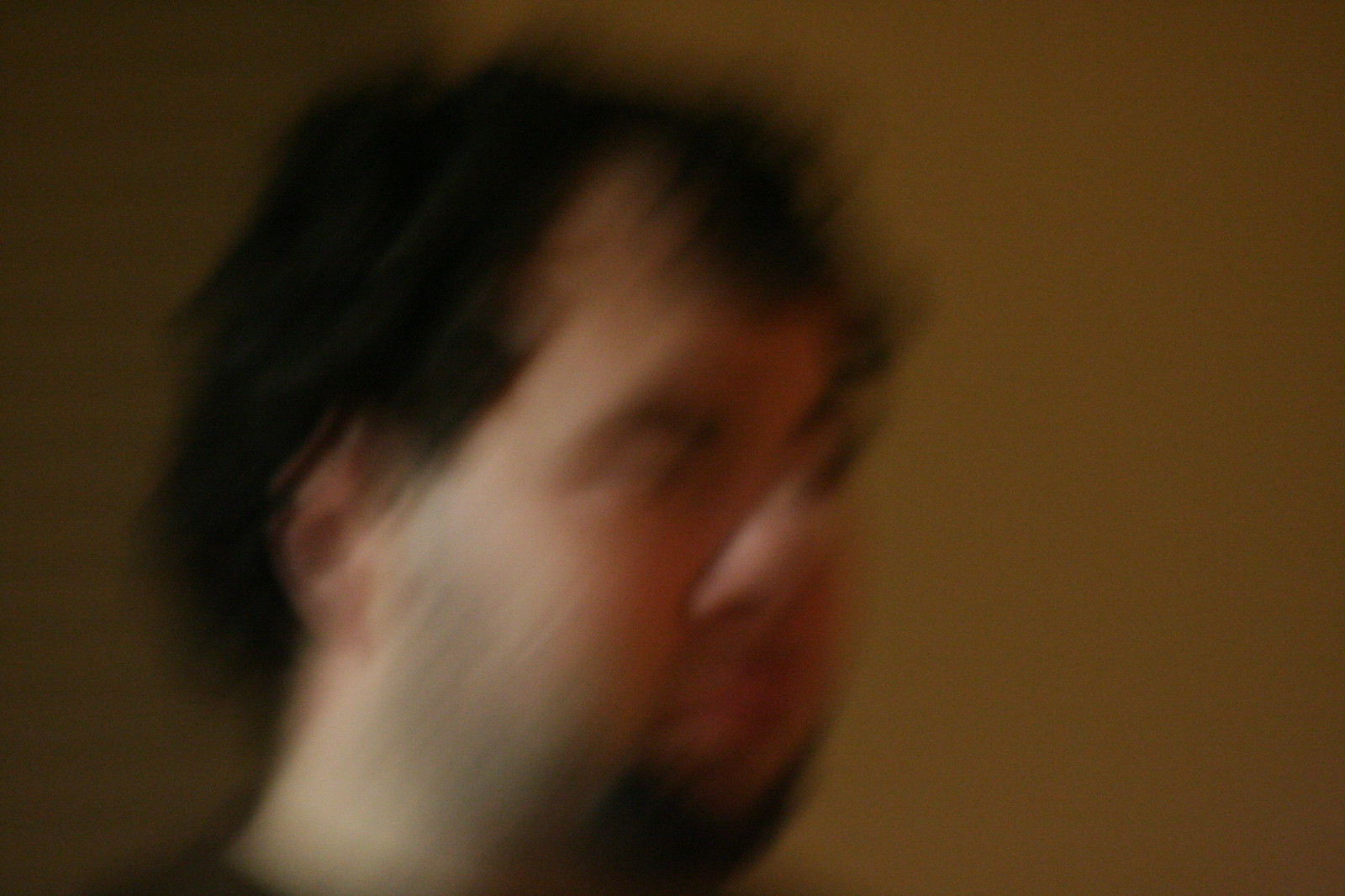The image depicts a very blurred figure of a man with light skin and dark, curly hair that falls just to the neckline. He appears to have a dark-colored goatee under his chin and dark eyebrows. Though his eyes are quite blurred, they seem to be dark-colored as well. There is visible stubble on the sides of his face, and his hair looks somewhat unkempt. He is wearing a dark-colored shirt or top, which can just be made out toward the bottom of the image before it crops out. The background features a gradient of dark brown, lighter on the right side than on the left.